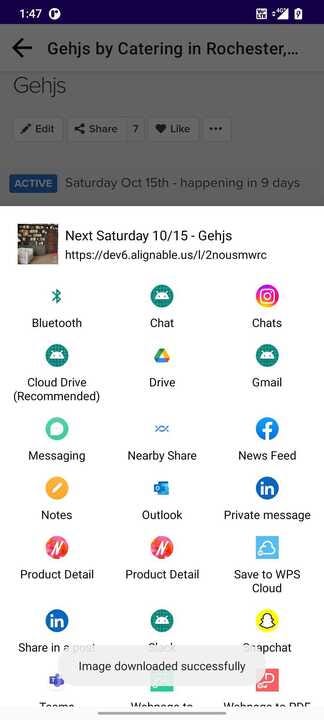**Screenshot on Mobile Device: Detailed Description**

This screenshot captures the user interface of a mobile device at 1:47 PM, evident from the time displayed in the upper left-hand corner. In the upper right-hand corner, icons for battery life and 4G network status are clearly visible. Below this status bar, the user has performed a search query for "gigs by catering in Rochester."

Just beneath the search bar, there are buttons for "Edit," "Share," and "Like." Further down, an upcoming calendar event is shown, detailing "Next Saturday, 10.5 gigs," followed by a URL. 

The bottom section of the screenshot features a grid of app icons categorized into five rows:

- **First Row:** Bluetooth, Chat, and Chats apps.
- **Second Row:** Cloud Drive Recommended, Google Drive, and Gmail (notably, the Gmail app here displays an Android logo instead of its usual icon).
- **Third Row:** Messaging, Nearby Share, and News Feed, which includes the Facebook logo.
- **Fourth Row:** Notes, Outlook, and Private Messages.
- **Fifth Row:** Product Detail, another Product Detail app, and Save to WPS.

Each icon is properly labeled with its respective app name, enabling easy identification and access.